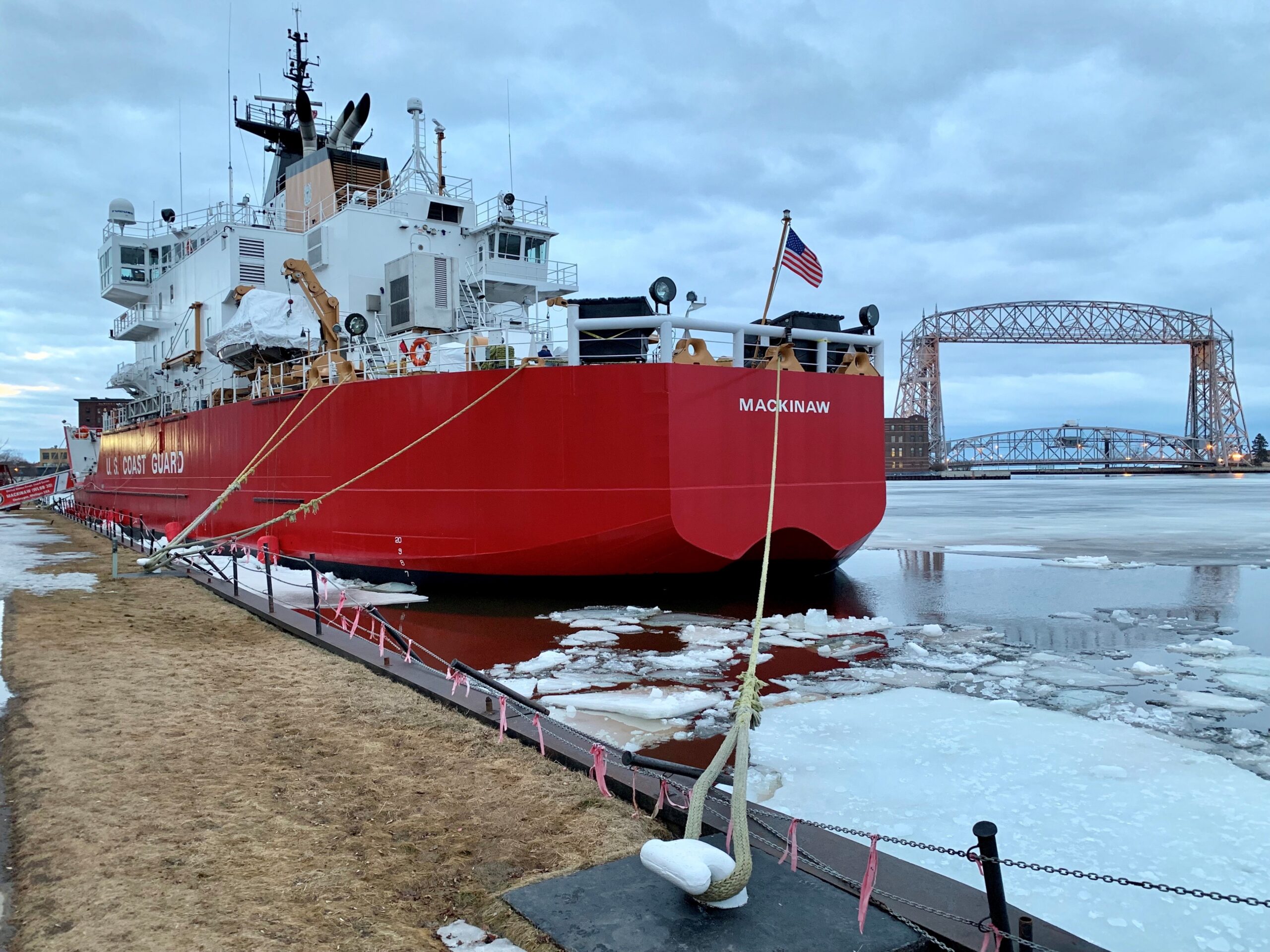This detailed photograph captures a large U.S. Coast Guard ship named Mackinac, prominently displaying the American flag. The imposing vessel, docked and tethered securely with substantial ropes, boasts a striking color scheme—red on the bottom and white on the top. The ship appears to have multiple rooms or compartments, indicative of its functional design. The cold water surrounding the ship is partially frozen, with sheets of ice of varying sizes floating on the surface. Additional ice and snow are visible on the ground next to the docked ship, contrasting with patches of brown grass. In the background, to the right of the ship, a bridge spans the scene under a cloudy, grayish-blue sky. The overall atmosphere suggests a cold, possibly wintery day with no people in sight.